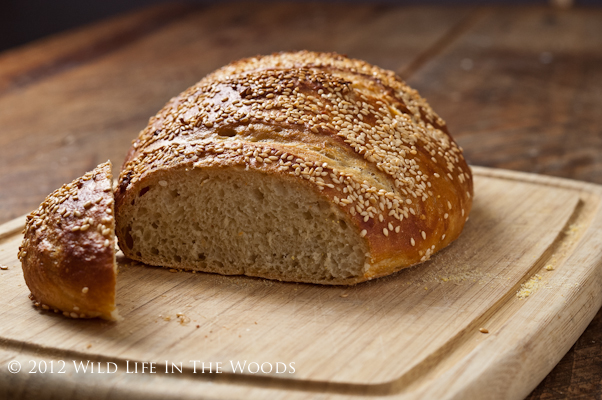The image features an oval-shaped loaf of wheat bread with white sesame seeds sprinkled on top. A single slice has been cut off from one end, revealing the bread's interior, which has small holes and a light tan color. The loaf is placed on a light brown, rectangular butcher block style cutting board. The board, accented with loose sesame seeds, rests on a darker brown wooden table or bench. The cut slice of bread is positioned catty-cornered to the front of the loaf. At the bottom of the image, the text "2012 Wildlife in the Woods" is visible, indicating the image's source or sponsor. The overall scene is a detailed, photographed depiction of freshly baked bread, emphasizing its texture and the contrasting wood tones.